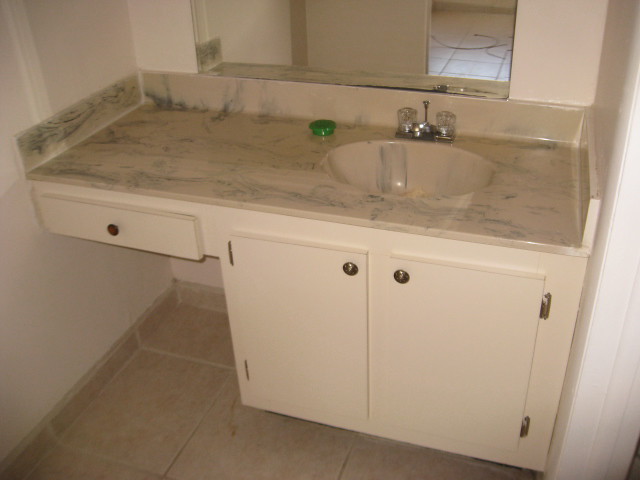This vividly detailed color photograph captures a bathroom vanity tucked into a niche, enclosed by white-painted walls on either side. The vanity features a single sink basin with a modest amount of the bottom half of a mirror visible above it. Reflected in the mirror is a floor of beige ceramic tiles with lighter colored grout. The vanity's countertop is white with elegant grayish-blue marble-like striations.

The polished chrome faucet is fitted with acrylic crystal knob handles, and the stopper is in the pulled-up position. To the left of the sink, a small, circular green dish rests on the countertop. Notably, the left side of the vanity has an open area beneath the countertop, suitable for placing a chair. Just above this open space is a drawer, adorned with a round, dark-colored handle.

In front of the sink basin, the vanity features two cabinet doors, each equipped with matching round handles, all painted in a pristine white. The overall design and color scheme of the vanity, along with the walls, contribute to a clean and unified aesthetic.